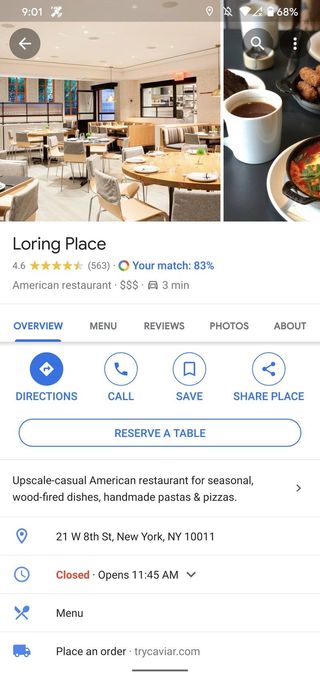A comprehensive review of the New York-based restaurant, Loring Place, is displayed on a smartphone with the battery life at 68% and the time at 9:01. The user interface includes a back button for navigation. The image portrays Loring Place as a very basic and down-to-earth restaurant, devoid of fancy decorations. The seating comprises simple chairs and tables without tablecloths, set against beige walls, creating a flat and unremarkable ambiance lacking in color or plant life. Despite the plain aesthetic, Loring Place boasts a commendable rating of 4.6 out of 5 stars and a personalized match of 83%. Categorized as an upscale casual American restaurant, it features three dollar signs indicating a moderate to high price range, and is conveniently located just three minutes away.

On the right side of the review, there's a partial image showcasing the food, including a cup of coffee, what appears to be mozzarella sticks, and an item in a sauce, suggesting an Italian influence. The bottom section of the screen provides navigation options such as Overview, Menu, Reviews, Photos, and About, with additional buttons for getting directions, reserving a table, calling ahead, saving, and sharing the listing. The description at the bottom highlights that Loring Place specializes in seasonal wood-fired dishes, handmade pastas, and pizzas.